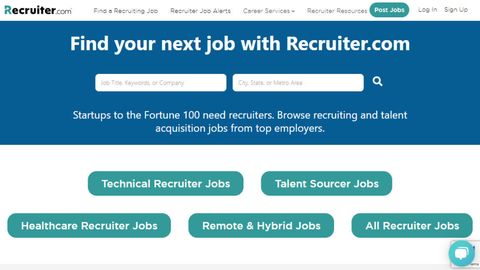This image, sourced from recruiter.com, features a user interface designed to assist individuals in finding recruitment-related jobs. The site provides several functional options, including "Find a Recruiting Job," "Recruiter Job Alerts," "Career Services," and "Recruiter Resources." A prominent green and white 'Post Jobs' button is visible, along with 'Log In' and 'Sign Up' options for users.

Central to the interface is a search tool that allows users to search for jobs by city, state, metro area, job type, keywords, or company. The platform promises opportunities ranging from startups to Fortune 100 companies, emphasizing the need for recruiters. Below this, there are several green and white buttons categorized by job types: "Technical Recruiter Jobs," "Talent Sourcer Jobs," "Healthcare Recruiter Jobs," "Remote and Hybrid Jobs," and "All Recruiter Jobs." Each button provides quick access to specialized job listings tailored to specific recruitment areas.